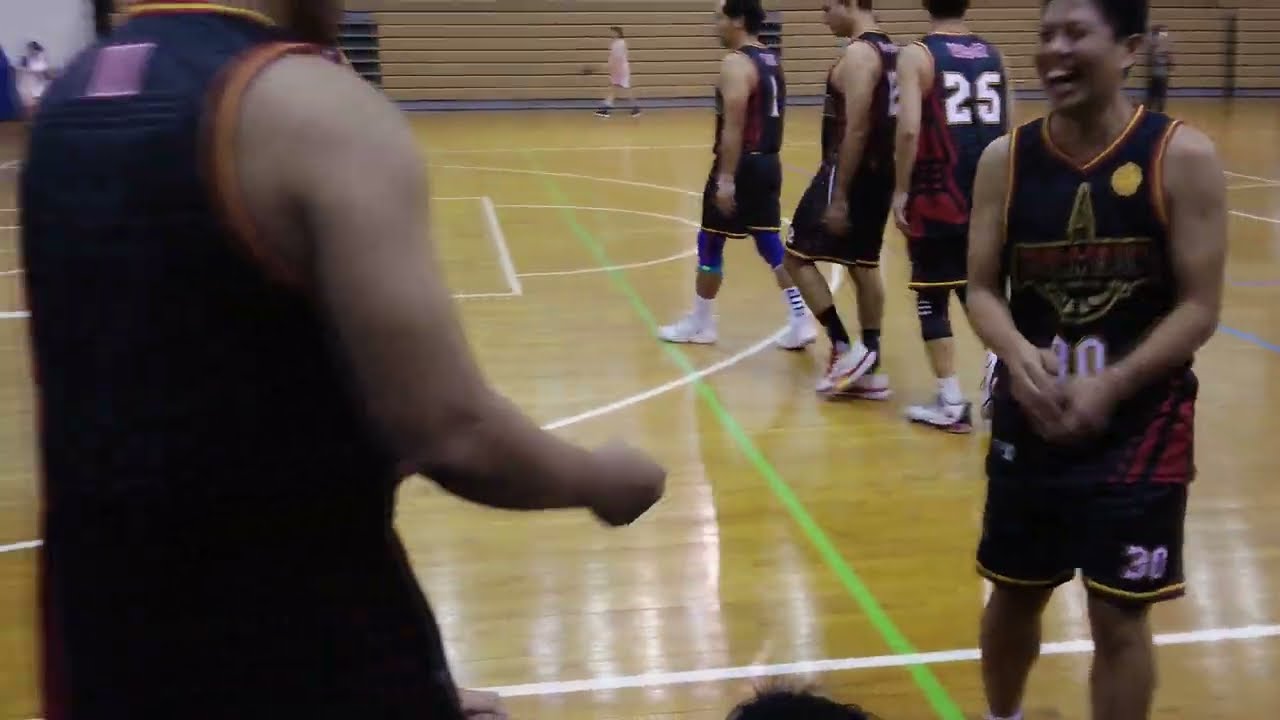The image shows an indoor, hardwood basketball court in daylight, characterized by lined markings for basketball, such as the white three-point line and free throw lane. The scene is populated by a group of basketball players in matching dark blue uniforms with white numbers and orange and gold edging. The players are walking and interacting, all wearing white athletic shoes. One player with the number 30, who is facing the camera and smiling broadly as if laughing, is engaged in conversation with another player whose back is to us. Other visible numbers include 1, 2, 12, and 25. The players appear to be of Asian descent and have brown skin. Wooden bleachers are collapsed against the far wall, and a few girls in white attire are spotted in the background. Additionally, another figure wearing white moves across the gym floor carrying something black. The image's composition is a realistic color photograph in landscape orientation.